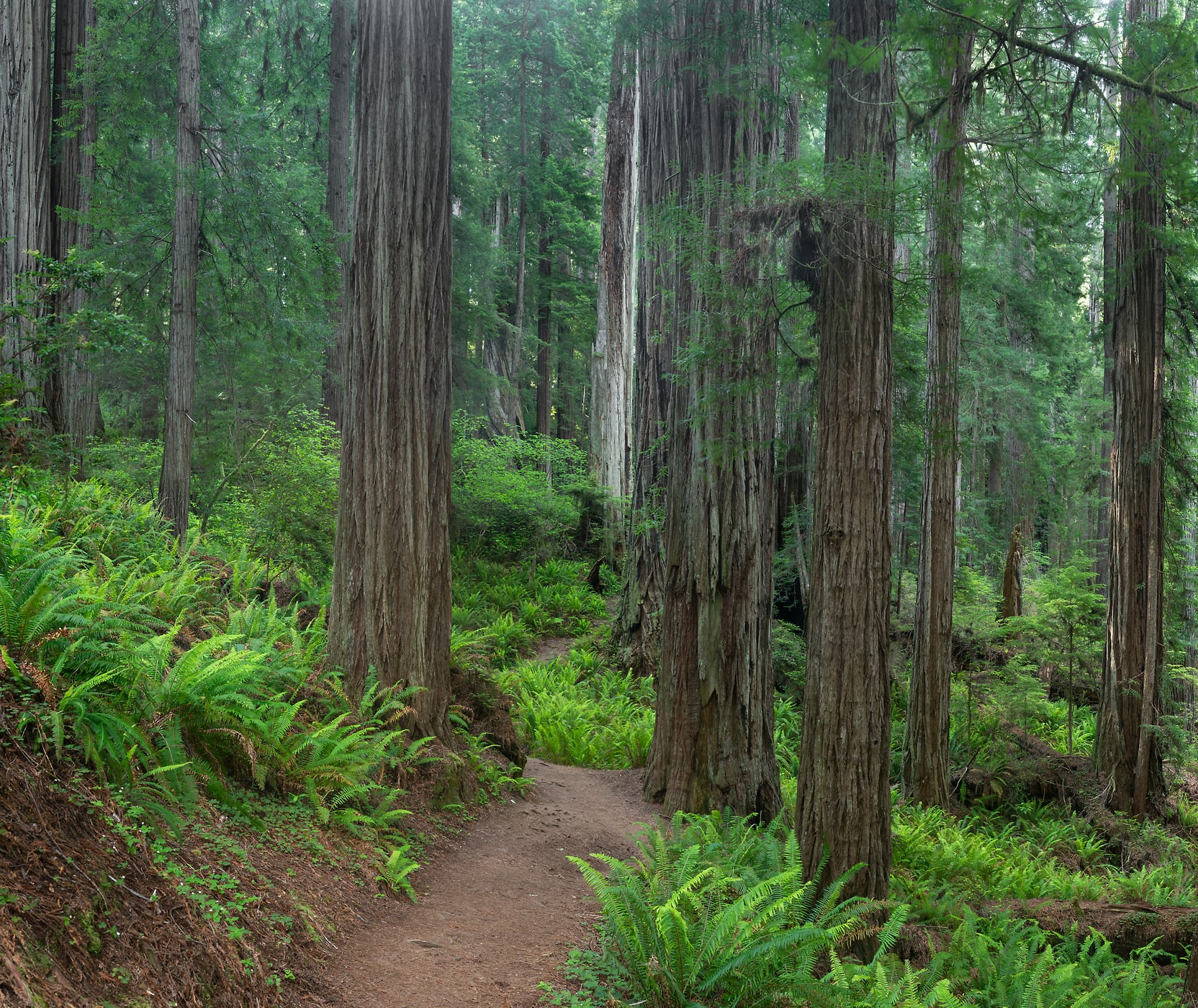The photograph captures an inspiring scene of a dense forest on a pleasant, rain-free day. You find yourself walking along a narrow, light brown dirt path that begins near the viewer and winds off into the distance. Towering cedar trees dominate the scene, distinguished by their tall statures, wide bases, and light brown to grayish bark, which appears scaly and papery. The forest floor is lush with green fern shrubs and other undergrowth, providing a rich, verdant contrast to the earth-toned path. Fallen trees, some covered in moss, add to the natural, untouched beauty of the setting. The dense canopy of leaves high above creates a closed, immersive environment, making the sky invisible. There are no humans or animals in sight, heightening the sense of pristine tranquility within this West Coast woodland, reminiscent of the areas around Seattle, Washington.